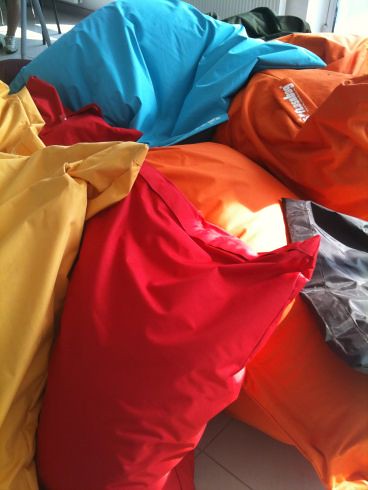This image captures a close-up, top-down view of a pile of multicolored objects, likely pillows or pillowcases with contents not fully filling them, making them appear wrinkled and smushed together. The colors visible, starting from the top and moving clockwise, are blue, orange, red, yellow, and light blue, with an additional red piece slightly obscured beneath the blue pillow. There's also a hint of a dark green or gray object resting on top of the blue and orange items. The scene is set against a white tile floor visible in the lower right corner, with darker grout lines separating the tiles. Sunlight casts across the pile from the right side of the frame, creating areas of light and shadow. In the upper left section of the image, partially out of focus, we can see the bottom of a person's leg, suggesting they are sitting down, with what may be chair or table legs around them. The background includes some white walls and potentially other furniture, adding context to the room’s indoor setting.